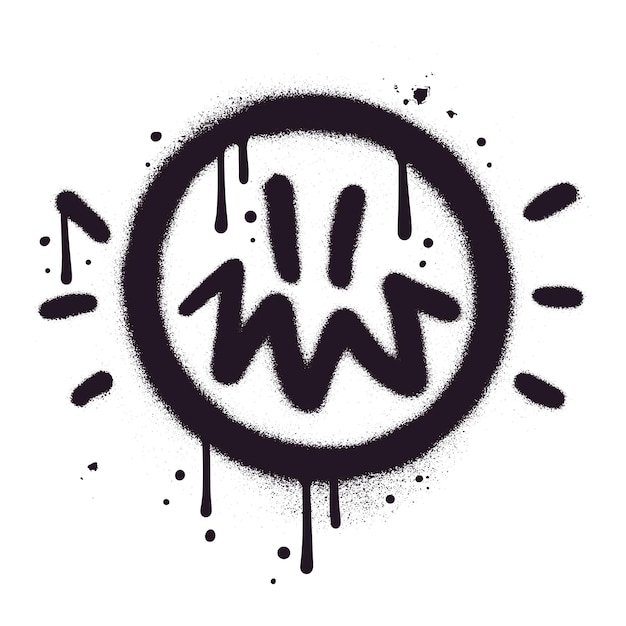The image is a simplistic black-and-white painting, likely created using either spray paint or an airbrush, as evidenced by the air-induced droplets and some runs in the paint. The composition features a central circle resembling a stylized smiley face, floating on a stark white background with no frame or text. The eyes are depicted as elongated vertical slashes, while the mouth is a jagged, squiggly line reminiscent of a jack-o-lantern, imparting a somewhat menacing expression rather than a cheerful one.

The face is framed by multiple paint drips—three inside the circle and three underneath—adding texture and variation to the otherwise smooth application. Additionally, the circular face is adorned with several dots, three on each side, mimicking rays or a sunburst effect that childlike drawings often feature. The periphery of the face is surrounded by smaller black dots of varying sizes, contributing to a fuzzy, almost furry aura around the circle, enhancing its visual intrigue.